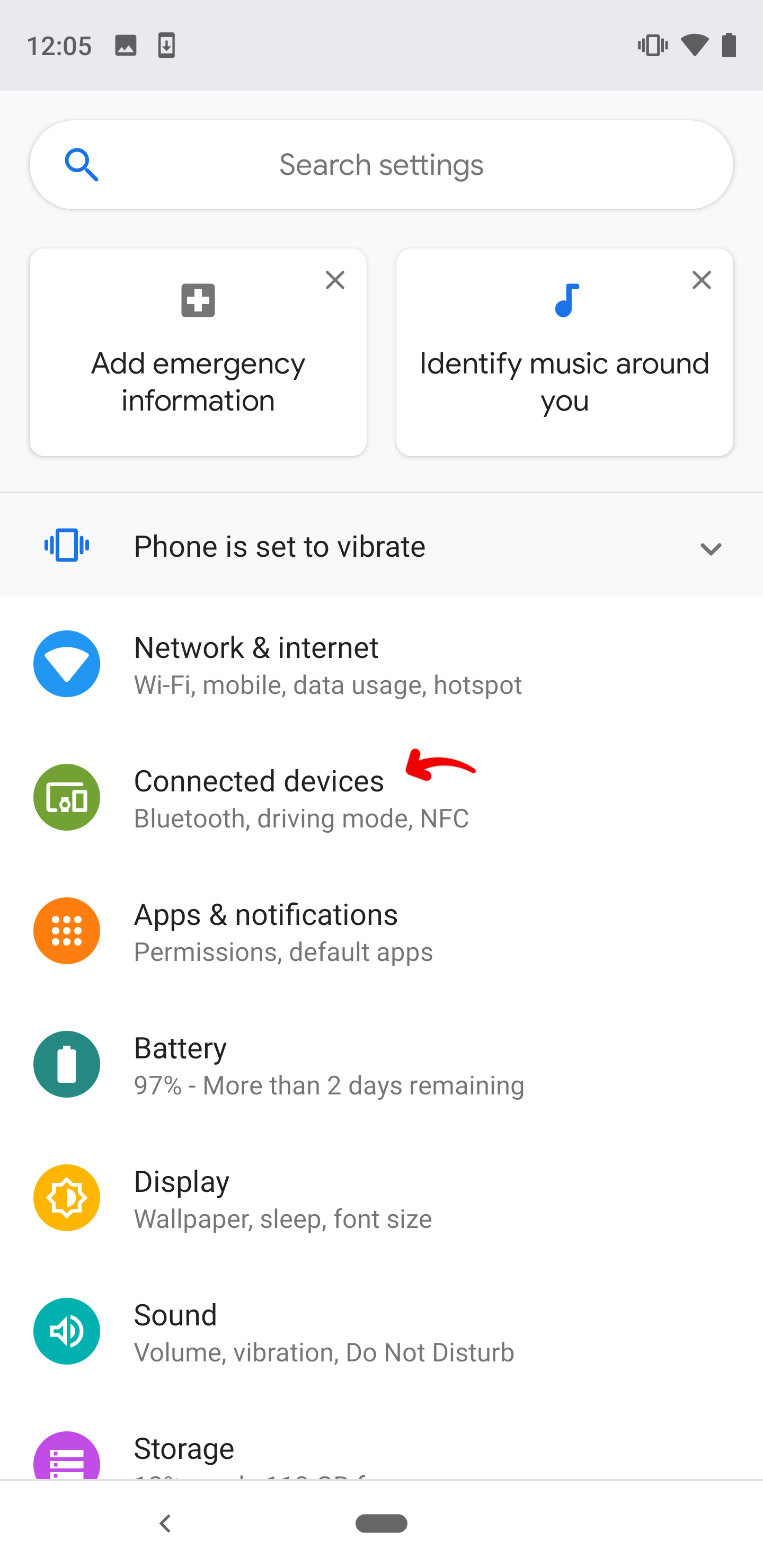This image appears to be a screenshot taken from an Android device, possibly a tablet or phone, showcasing the settings menu. 

At the very top, there is a light gray toolbar. On the top left, it displays the time "12:05". Adjacent to this, there are icons for the gallery and a software download indication (a small screen with a downward arrow). On the far right side of the toolbar, icons indicate that the device is on vibrate mode, the Wi-Fi is fully connected, and the battery is fully charged.

Below this toolbar, a search bar is prominently displayed with the text "Search settings." Immediately below the search bar, there are two interactive text boxes. The first box, featuring a white plus sign within a gray square, prompts the user to "Add emergency information." Next to it, a blue music note icon suggests the option to "Identify music around you."

Following these options, there is an icon of a phone set to vibrate accompanied by the text "Phone is set to vibrate." Below this, several settings categories are listed:

1. **Network & Internet:** Represented by a blue circle with a white Wi-Fi icon, this section includes options for Wi-Fi, mobile data usage, and hotspot.
2. **Connected Devices:** Indicated by a green circle with an icon of connected devices in white, this section covers Bluetooth, drive mode, and NFC. Notably, there is a red arrow on the screen pointing towards this category, highlighting its current selection.
3. **Apps & Notifications:** Marked by an orange circle with nine white dots, this menu handles permissions and default apps.
4. **Battery:** Shown by a turquoise circle with a white battery icon, it indicates that the battery is at 97% with more than two days of usage remaining.
5. **Display:** Represented by a yellow circle with a sun icon, this option includes settings for wallpaper, sleep, and font size.
6. **Sound:** Identified by a light blue circle with a speaker icon, it manages volume, vibration, and do not disturb modes.
7. **Storage:** The last option, displayed with a purple circle featuring three white files, pertains to storage management.

Each icon and description efficiently categorizes the various settings available on the Android device, providing a detailed and user-friendly navigation experience.